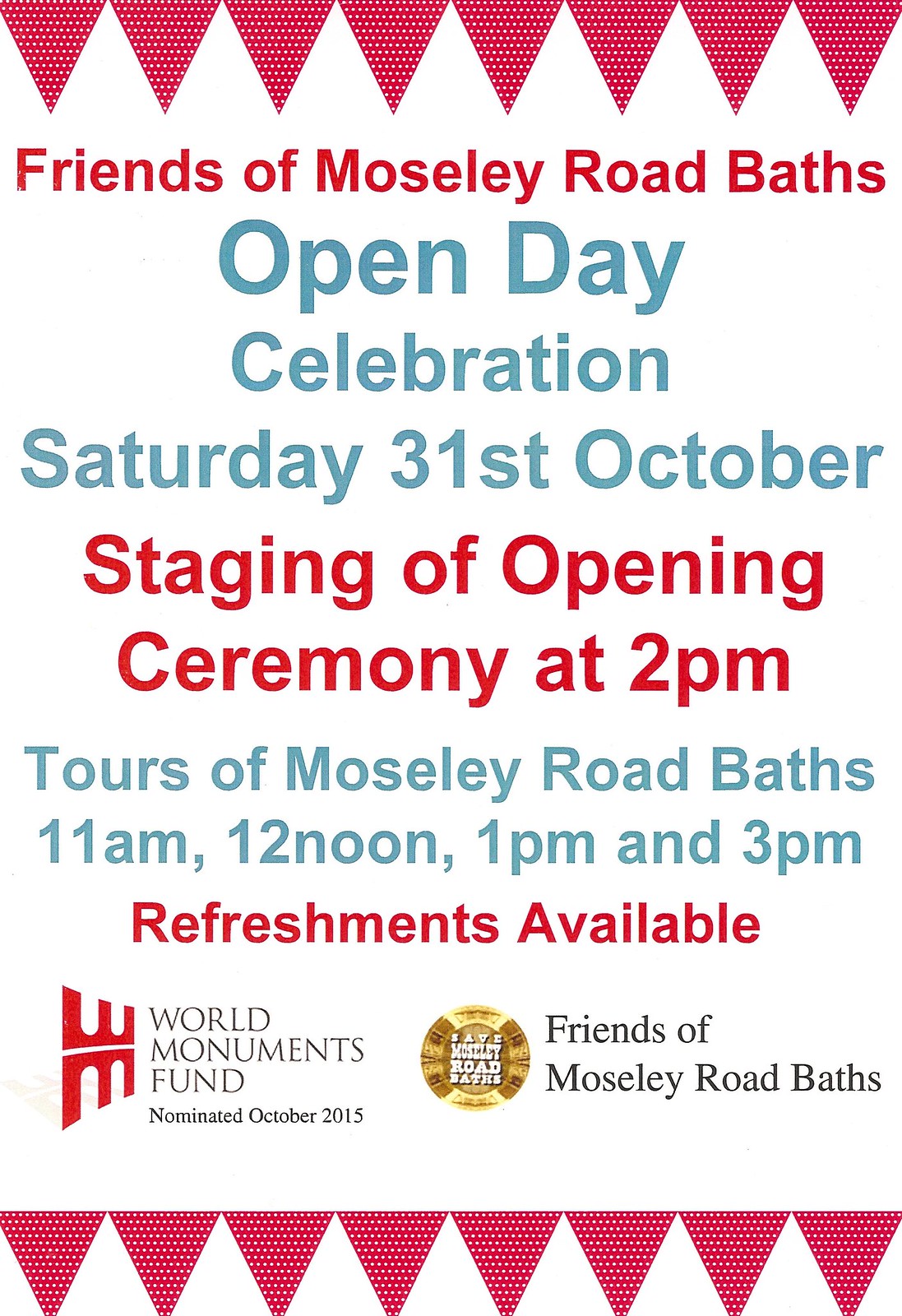The poster features a clean, white background adorned with vibrant text in red and blue. At the top and bottom of the poster, a design of red triangular flags adds a festive touch. The headline reads "Friends of Mosley Road Baths" in red, followed by a blue subheading announcing the "Open Day Celebration" on "Saturday, 31st October." Specific event details are listed below: "Staging of Opening Ceremony at 2pm" in red, and "Tours of Mosley Road Baths at 11am, 12noon, 1pm, and 3pm" in blue, along with a note in blue that "Refreshments Available." For additional context, the poster includes two logos at the bottom—one on the left in red for the "World Monuments Fund," which notes the nomination in "October 2015," and another on the right, a yellow circular logo representing the "Friends of Mosley Road Baths." The overall design is neatly structured with repeating elements to maintain a cohesive and inviting aesthetic.